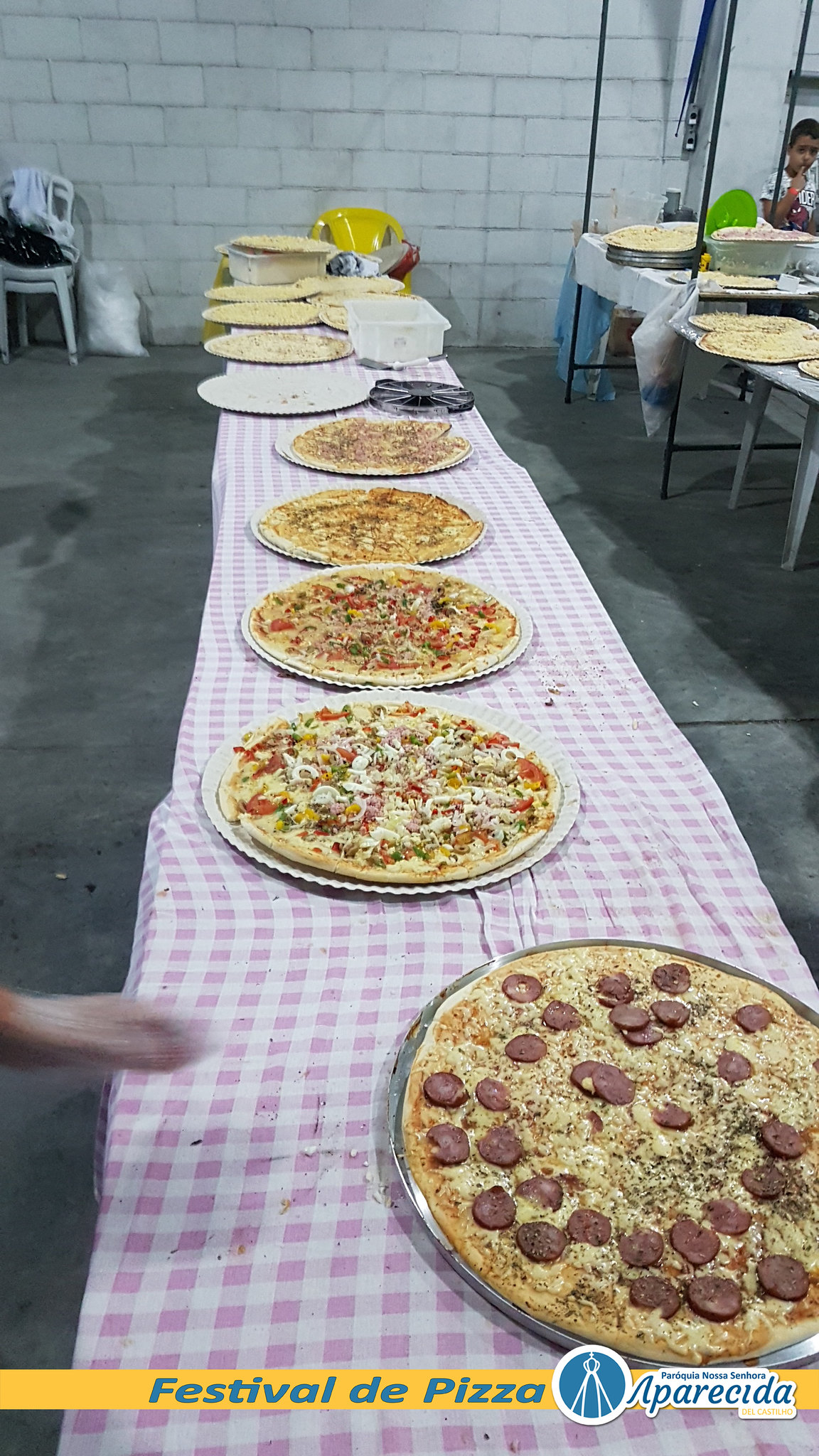This vibrant color photograph captures a festive scene of a pizza feast set along a seemingly endless banquet-style table covered in red and white checkered tablecloths. The table boasts a variety of pizzas, including pepperoni, bell pepper, sausage, and cheese, as well as others adorned with various vegetables and meats. In the background, a child stands near more tables, perhaps involved in the cooking process, with his finger thoughtfully to his mouth. The setting appears outdoors, with a gray concrete floor and a brick wall at the back adding a rustic charm. Toward the front of the image, a blurry hand reaches for a slice, emphasizing the communal nature of the feast. The photograph is part of the "Festival de Pizza, Aparecida, Parroquia Nossa Senhora," as indicated by the text at the bottom, celebrating the joy of shared pizza in a warm, community-centric environment.